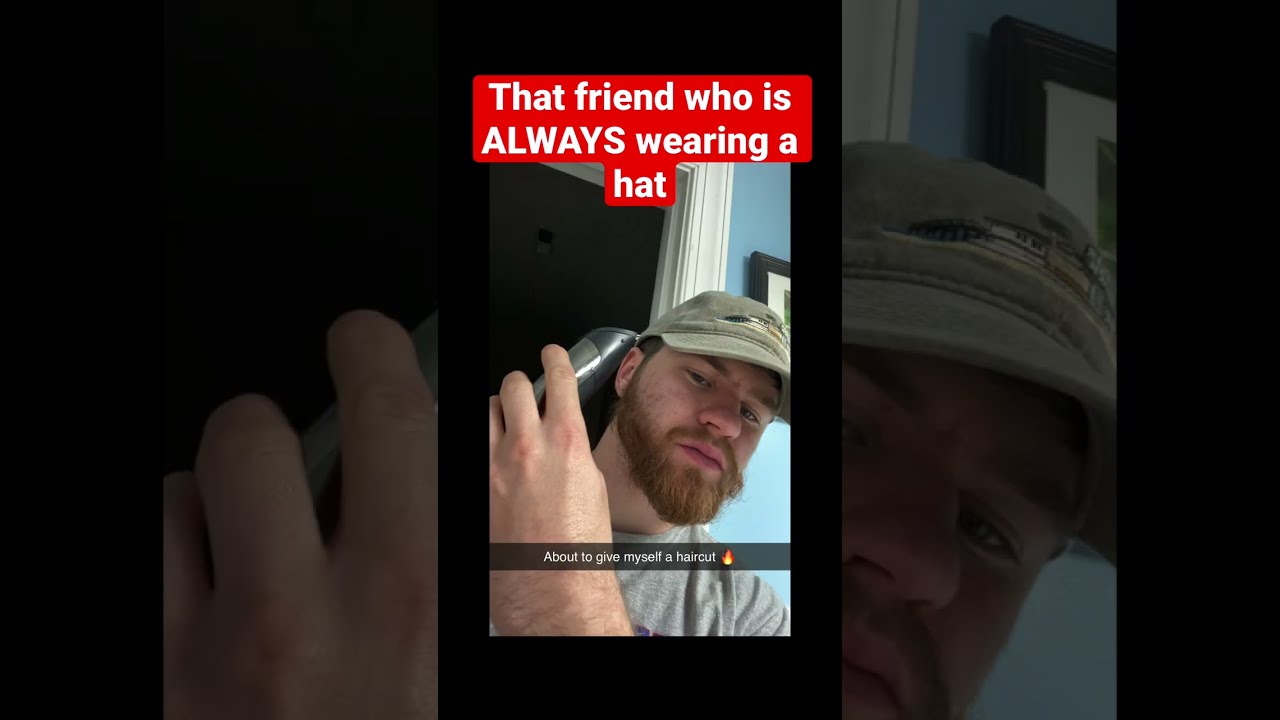The image features a selfie-style portrait of a white man with a full brown beard and mustache, slightly reddish in tone. He is wearing a gray baseball cap with a brim nearly level with his eyebrows. The man holds an electric razor up to his left ear, appearing ready to give himself a haircut. His expression is rather blank as he looks slightly down at the camera. The background features an open door with a white trim leading to a blue wall on the right. A picture frame with a dark wooden motif hangs above his hat on this blue wall. The image includes text overlays: above the man’s head on a red background with white lettering, it reads, “That friend who is ALWAYS wearing a hat,” with "ALWAYS" in all caps. At the bottom, a semi-transparent dark gray bar contains the text, “About to give myself a haircut,” alongside an image of a flame icon. The image is vertical with tinted and zoomed-in sections of the central picture on both sides.